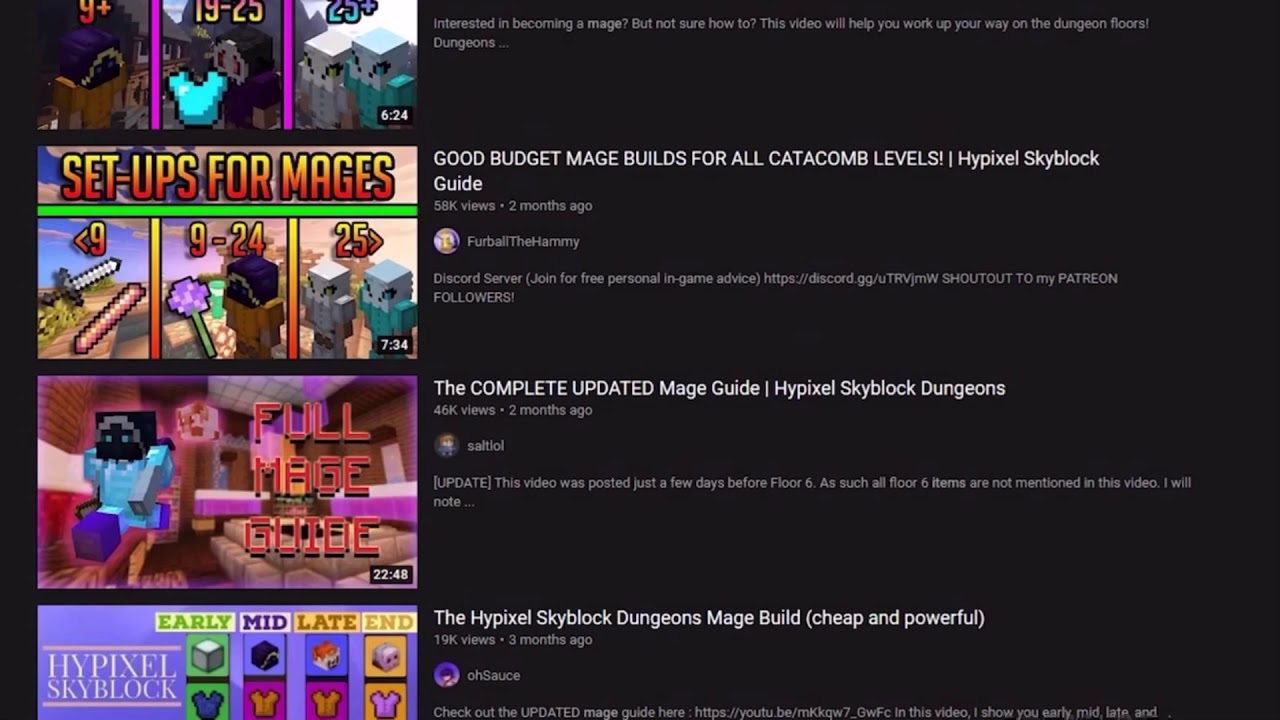This is a web page on a gaming website, dedicated to providing game guides and information. The page features several images on the left side, clearly related to the content for various games. The first image showcases characters resembling robots and contains the text "9+, 9-25, and 23+", along with a time stamp at the bottom that reads "6-24". Below these images, there is an orange text header that reads "Setups for Images," next to what appears to be a sword icon.

The first setup image features a backwards-facing arrow and the number 9 in orange letters. The second image displays a robot with the notation "9-24". The third image shows two robots with the numbers "25" and a right-facing arrow. Additionally, there is an image beneath these that depicts a robot in action with the text "Full Maj Guide," indicating a duration of "22 minutes and 48 seconds." The last image in this series reads "Early, Mid, Late, End" over blocks containing various images, all under the heading of "High Pixel Skyblock" (where "High Pixel" is one word).

On the right side of the page, there is a black background with white text. It begins by referencing the top three images and asks, "Interested in becoming a Mage (M-A-G-E), but not sure how to?" It continues to promise helpful video instructions for progressing through the dungeon floors. Further down, there are several headings: "Good Budget Mage Builds for all Catacomb Levels. High Pixel Skyblock Guide," followed by "Complete Updated Mage Guide. High Pixel Skyblock Dungeons," and "High Pixel Skyblock Dungeons Mage Build - Cheap and Powerful."